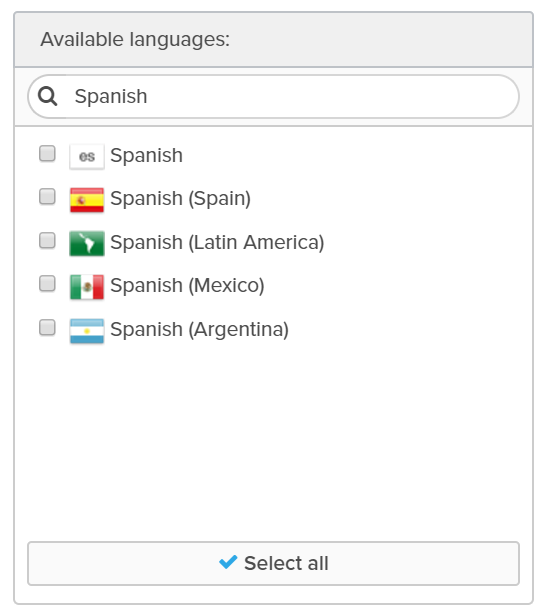The image appears to be a screenshot from a larger display, possibly a desktop or tablet, though it's cropped to hide identifiable browser or operating system elements. At the top, there's a pale gray header with black text reading "Available Languages." Below this header, a search bar is present, containing the already-searched term "Spanish." 

Beneath the search bar, a list of search results is displayed. Each result features a checkbox on the left, all currently unchecked, accompanied by a representative flag and the corresponding variant of Spanish. 

- The first entry features a plain white flag with "ES" text, labeled simply as "Spanish."
- The second entry displays a red and yellow flag, labeled "Spanish (Spain)."
- The third entry shows a green-colored flag with a map graphic, labeled "Spanish (Latin America)."
- The fourth entry features a flag in green, white, and red, labeled "Spanish (Mexico)."
- The fifth entry has a blue and white flag, labeled "Spanish (Argentina)."

At the bottom of the list, there's an option to "Select All," or users can choose to check individual boxes next to each variant. The layout and functionality suggest that this screenshot is from an application or website allowing users to choose different variants of the Spanish language.